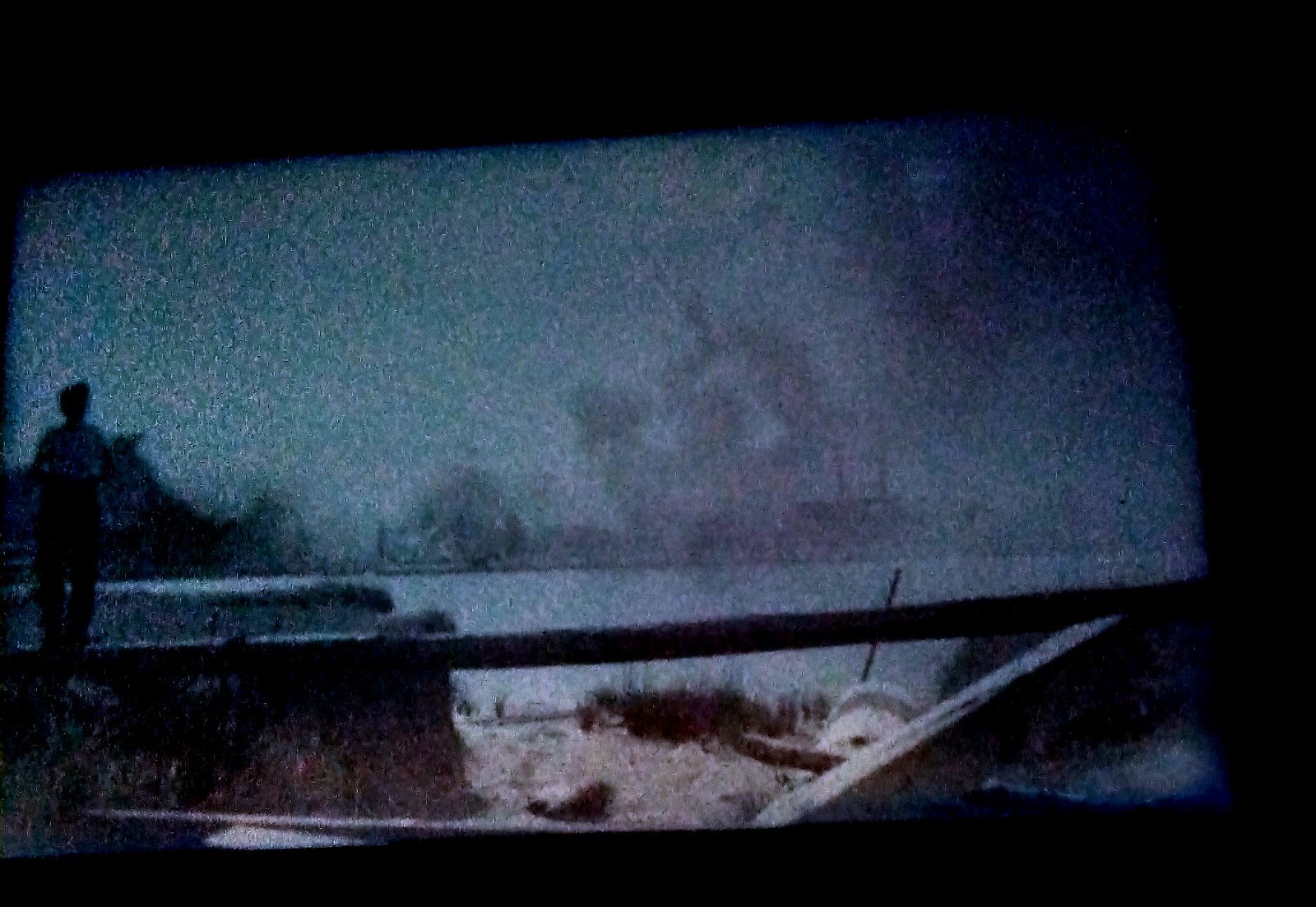The image presented is a very blurry, possibly painted, scene depicting a hazy beach or wasteland area during daytime. In the foreground, there's a silhouetted person walking towards the viewer from the left side. On the right side of the image, you can see some sandy terrain scattered with sticks and small plants. There appears to be a dry gully cutting through this wasteland, spanned by a log, possibly used to traverse the gully when it’s full. This gully contains various debris including a bucket, a big rock, and some grass. 

In the background, we observe a vast body of water, likely a lake or stretch of sea, with another potential individual standing at a distance near the shoreline. Across the water, the horizon showcases dark clouds or possibly smoke rising, hinting at pollution from what seems to be industrial buildings on the opposite bank. The overall color palette includes dark blues, teals, purples, greens, and pinks, contributing to the very dark, hazy atmosphere that obscures finer details of the scene.